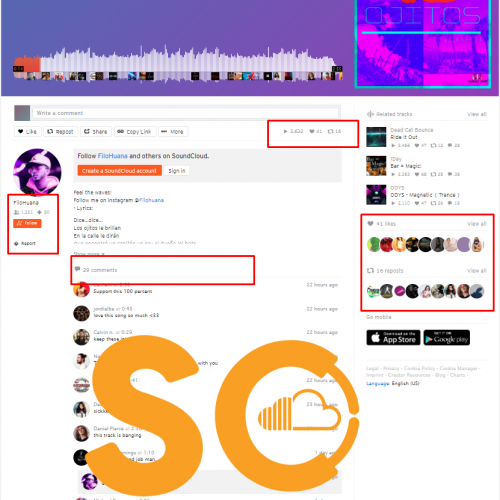This image depicts a SoundCloud page with several detailed elements. Across the top is a purple border adorned with indistinct, blurry images. In the top right corner, there's a slightly transparent rectangle with text that's difficult to read, though it ends with "TOS." The background of this area features predominantly pink and blue hues. 

Beneath this is a search bar with the faint text "write a comment." Next to it are options labeled "Selected Tracks" and "View All." Directly beneath the search bar is a heart icon followed by the word "Like." Adjacent to this are two arrows forming a loop, indicating the "Repeat" function, followed by "Share," "Copy Link," and "More" options. 

Further to the right, a prominent red-bordered play button is displayed with numerical indicators for plays, likes (represented by a heart), and shares (denoted by two arrows). 

Below these controls is a circular image of a man wearing a cap. Accompanying this image is the text: "Follow Filo, Juana, and others on SoundCloud. Create a SoundCloud account. Sign in." 

Additionally, there's some indistinct text mentioning "feel the waves follow me on Instagram," followed by lyrics. 

The bottom section displays "29 comments" with a red border. The page is superimposed with large text reading "SO", where the 'O' contains the SoundCloud logo.